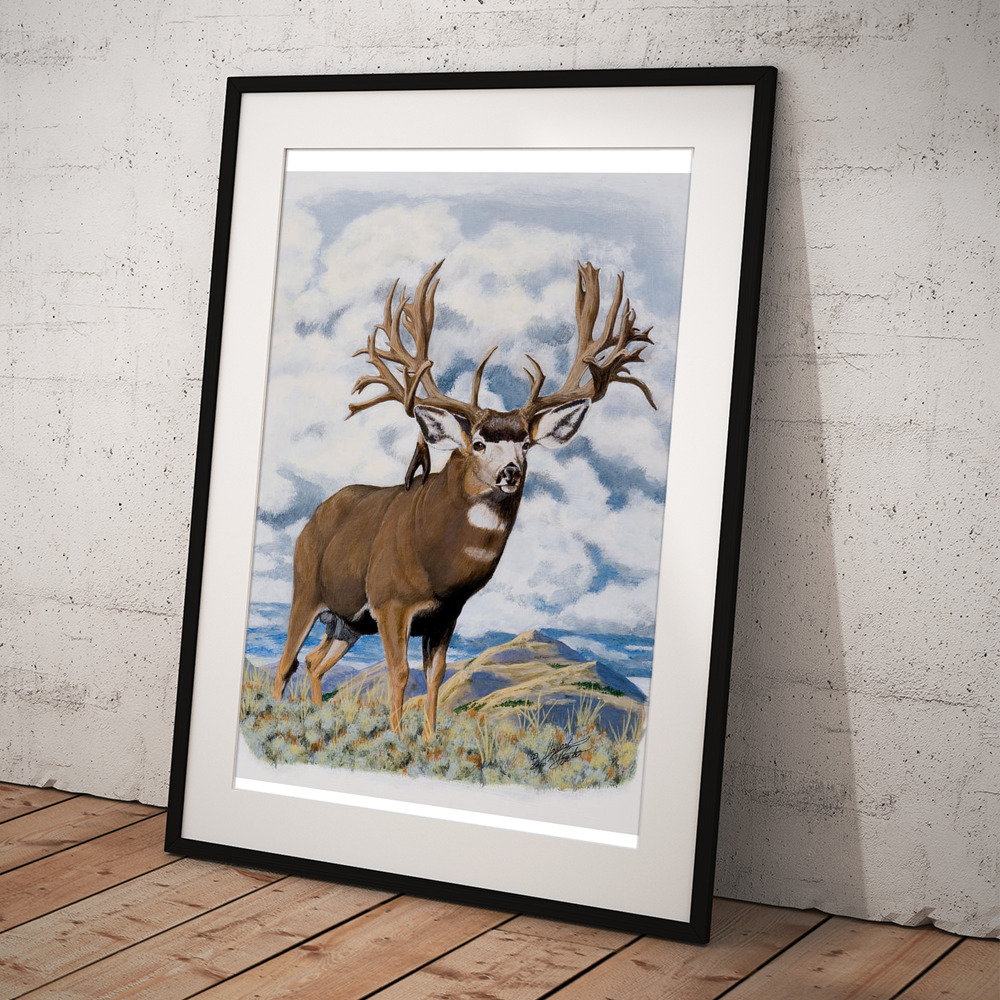This image depicts a large framed painting of an elk resting against a white, painted wall that shows signs of wear. The painting itself is set within a narrow black frame bordered by a thicker white matte. The elk, standing prominently in the foreground, is predominantly brown with a bit of white around its throat and face, and it boasts extensive antlers. The background features a mountain range, dry grass, rocky terrain, and a sky filled with white clouds. The frame sits on a wooden plank floor with the planks extending leftward and downward.